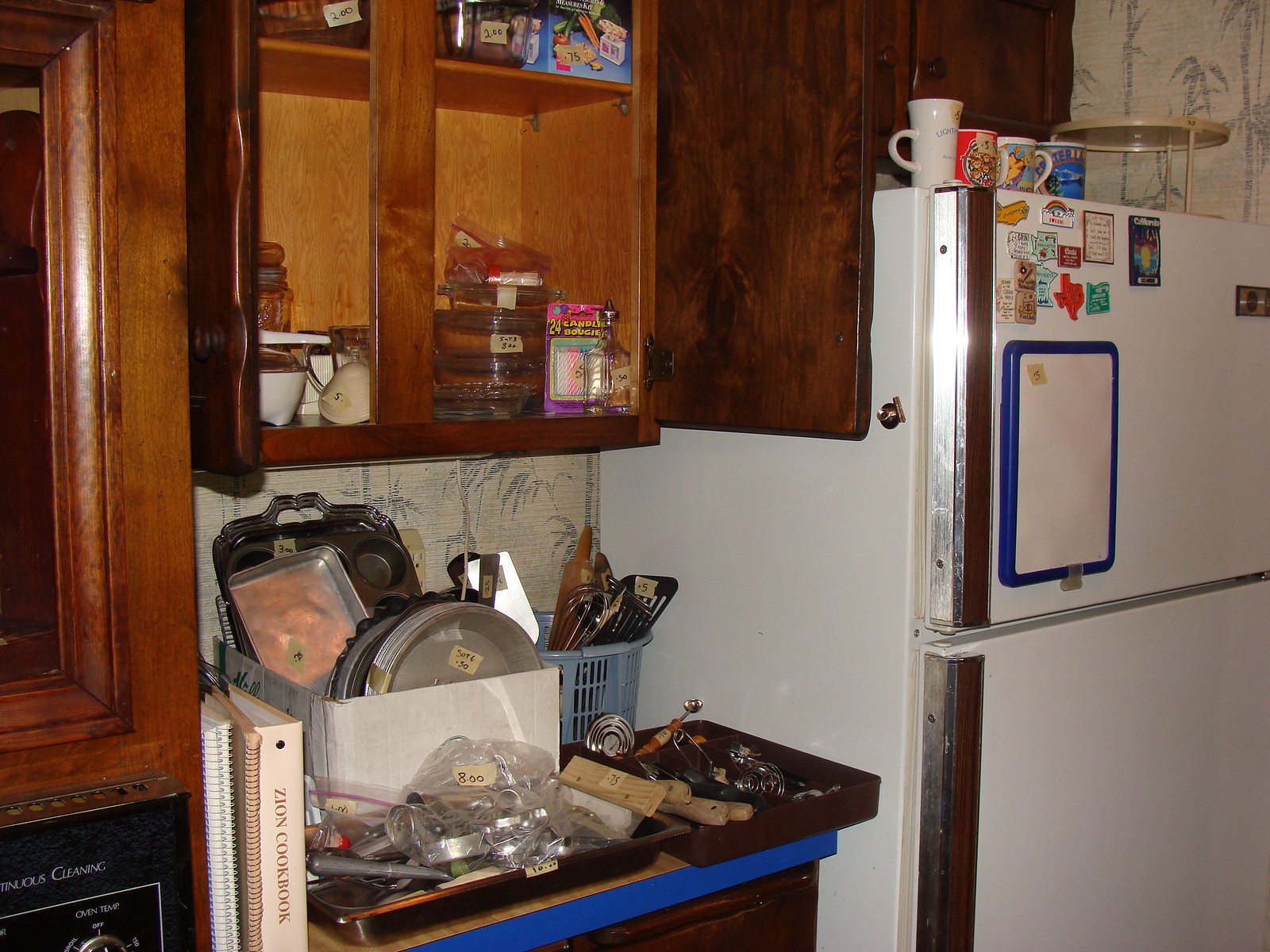This image captures a cozy, well-used kitchen with a white refrigerator prominently positioned on the right side. The refrigerator features a top freezer adorned with various magnets and a dry erase board for notes. Atop the fridge, there are several mugs and a glass pie saver, presumably for displaying baked goods like cookies, pies, or cakes. The appliance is snugly fitted within a wooden cabinetry setup, with two storage cupboards above it.

To the left of the refrigerator, a window allows natural light to filter into the room. Below this window sits a microwave, identifiable by its distinct knobs. Adjacent, a set of open cabinets reveals an assortment of dishes and food items, showcasing a blend of practicality and accessibility.

The kitchen countertop beneath the cabinets is scattered with a variety of kitchenware, including cookbooks, pans, and utensils, all of which hint at a space that is frequently used for home-cooking and culinary projects.